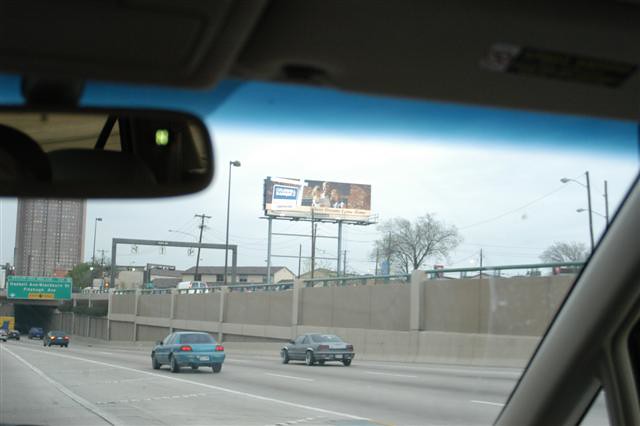This photograph captures the view from the perspective of a person looking out through the windshield of a moving car on a freeway. The top portion of the image includes a glimpse of the car's roof and sunshield, with the rearview mirror partially seen on the left side. The lower right corner reveals a small section of the passenger side metal frame beside the windshield. 

Through the windshield, the car appears to be in one of the left lanes of the freeway. Ahead, several vehicles occupy the right lanes: a blue car in the closest lane, an older gray car to its right, and another vehicle far in the distance below a green freeway exit sign. Above these cars, a towering skyscraper dominates the scene, accompanied by low-rise buildings to the right behind a roadside barrier. The sky has a hazy blue quality, and the distant horizon is dotted with power lines, a large billboard, and a couple of barren trees.